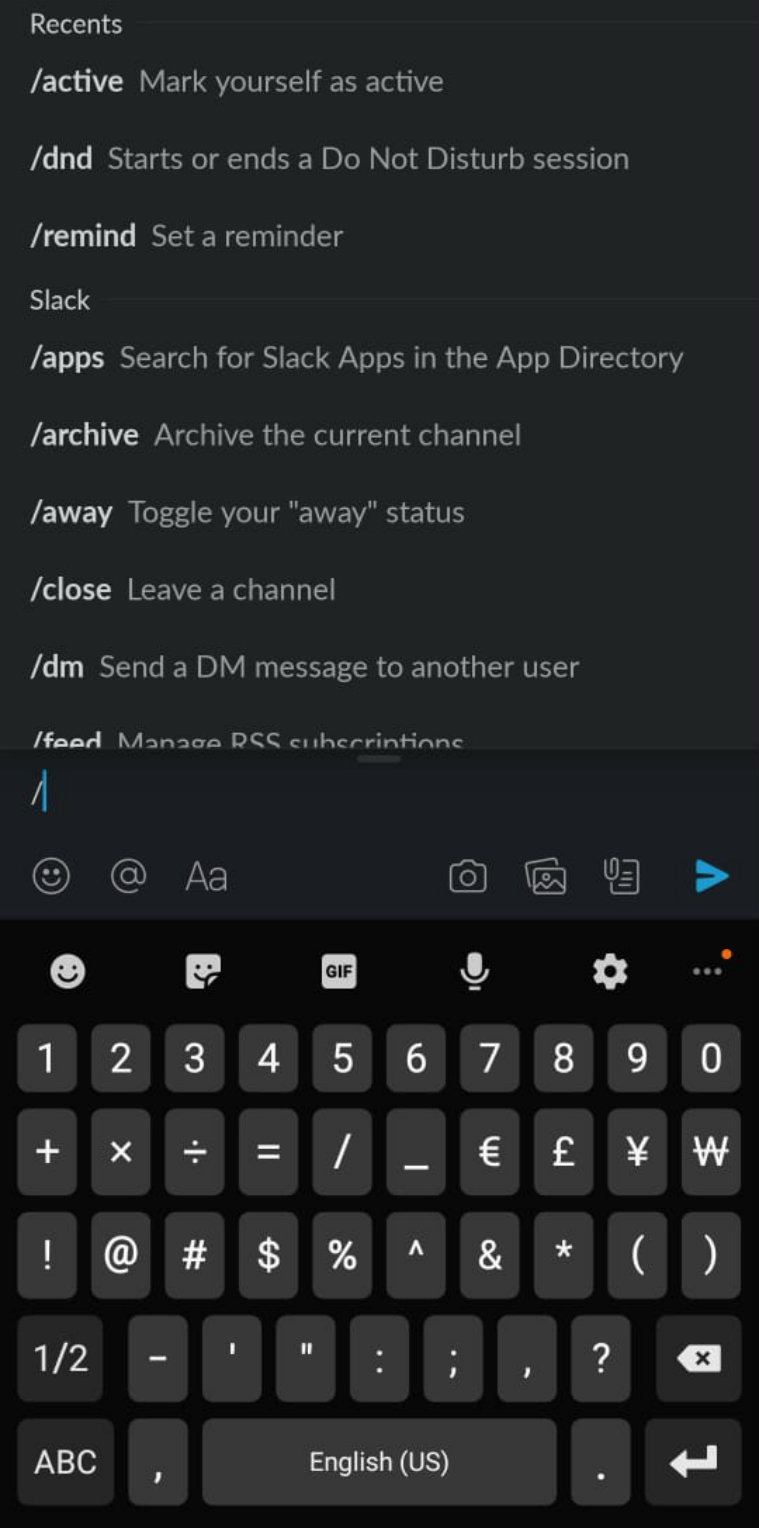In this image, we see a screenshot displayed against a solid black background. Beginning from the top left corner, there is a series of Slack commands listed in white text. Each command is accompanied by a brief description of its function. 

1. **/active** - Marks yourself as active.
2. **/DND** - Starts or ends a "Do Not Disturb" session.
3. **/remind** - Sets a reminder.
4. **/apps** - Searches for Slack apps in the app directory.
5. **/archive** - Archives the current channel.
6. **/away** - Toggles your away status.
7. **/close** - Leaves a channel.
8. **/DM** - Sends a direct message to another user.
9. **/feed** - Manages RSS subscriptions.

Towards the bottom of the list is a command represented as **/**, distinguished by a vertical blue line immediately below it. The commands are presented in a clear, organized manner, making it easy to understand their purposes.